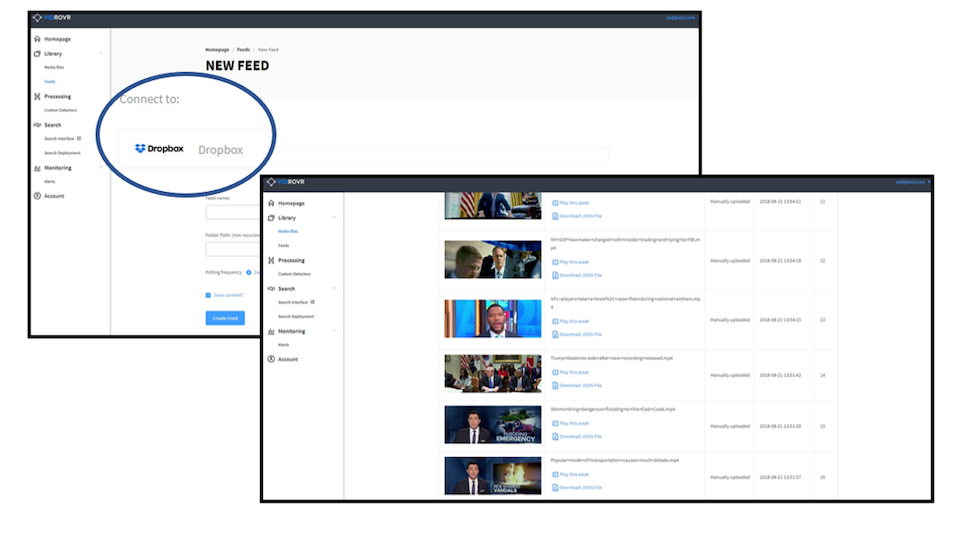The image displays two black interface screens from a platform called "Vic Rover." The screen positioned at the back prominently features a dark navy blue banner that reads "Vic Rover." This screen appears to be a Dropbox connection interface, with the Dropbox section highlighted and circled in blue. Multiple options are accessible via a column on the left side, including links to the homepage, library, processing, search functionalities, monitoring tools, and account settings. At the bottom of the screen, there is a login form requiring a username and password, accompanied by a blue login button.

Layered over the first screen is a second Vic Rover interface. Similarly, it includes the same left-hand column with navigation links to the homepage, library, processing, search features, monitoring tools, and account settings. The focal point of this screen is a collection of picture thumbnails, seemingly showcasing various individuals who might be news anchors or politicians. Some images appear to come from the White House, and one particularly resembles Donald Trump. Each thumbnail includes additional details such as dates, brief descriptions, and presumably links for playing or downloading the clips. Despite the wealth of information, the text on this screen is blurry and difficult to discern clearly.